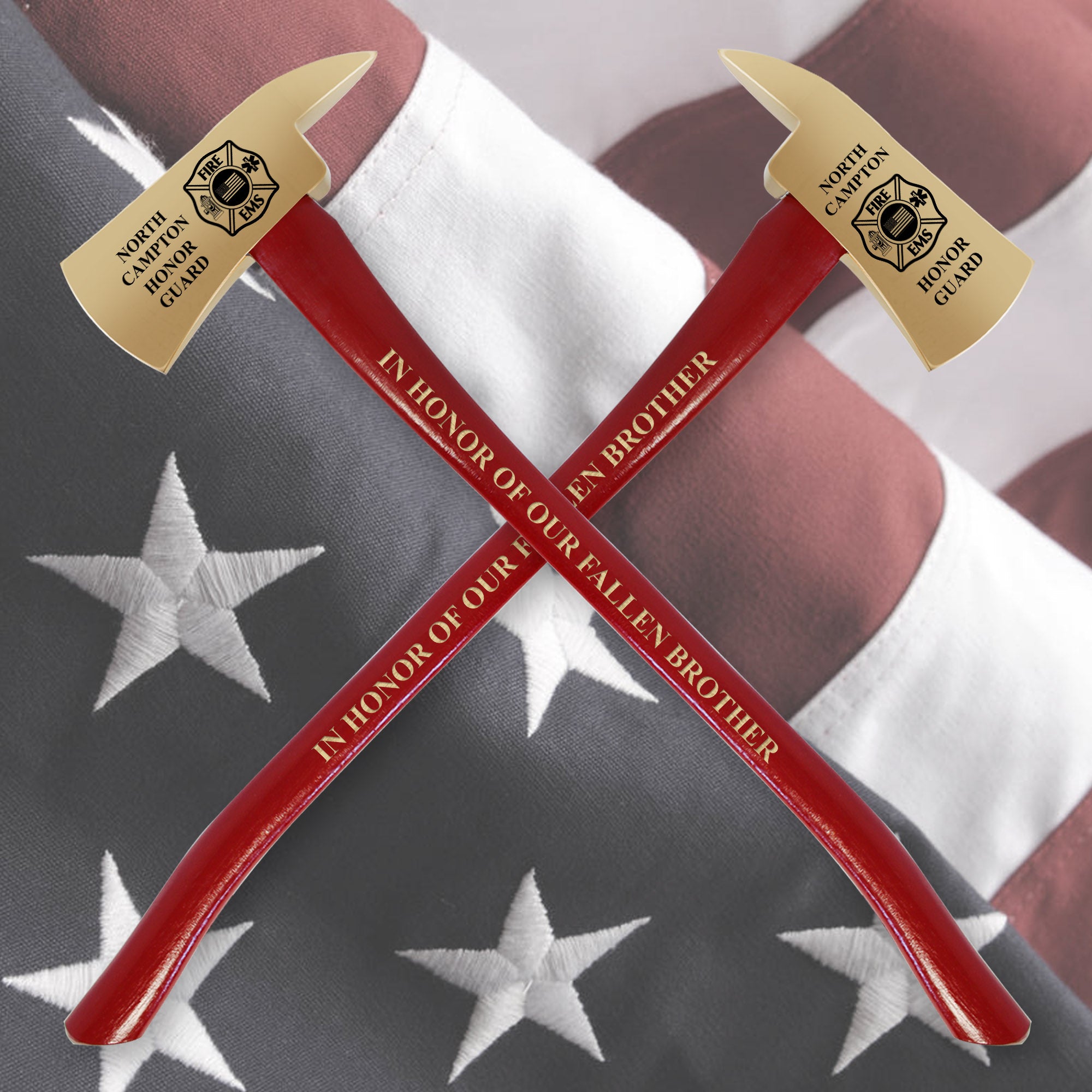This is a detailed image showcasing a somber tribute. The background is a slightly faded and folded American flag, with the blue field with white stars positioned diagonally from the lower left to the upper right of the square frame. In the foreground, two fire axes with red handles and gold blades are crossed to form an X shape. Each handle is inscribed with the text "In Honor of Our Fallen Brother" in gold. Each axe head bears the black text "North Campton Honor Guard" along with a detailed emblem. The emblem features a black circle with an American flag at the center, encircled by a gold ring labeled with "Fire" at the top and "EMS" at the bottom, flanked by two small, indistinct symbols. The interplay of colors—red, gold, black, white, and blue—and the detailed inscriptions convey a powerful and respectful homage to a fallen hero.